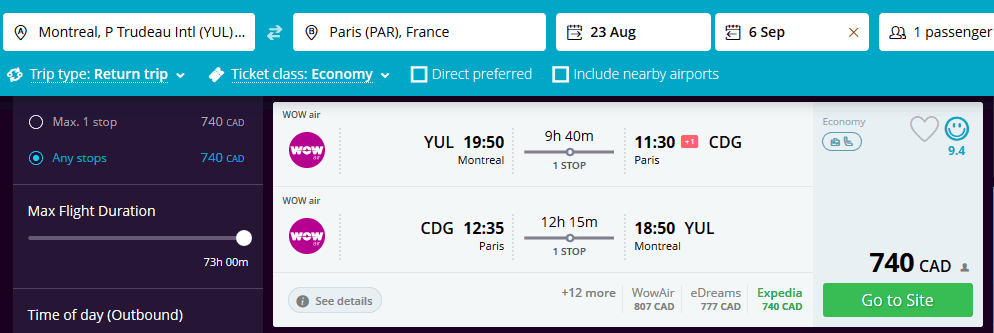The image appears to be a travel search page, likely for flights from Montreal P. Trudeau International (YUL) to Paris (PAR) in France. The page features a blue banner at the top with several white boxes. The first box indicates the departure location as "Montreal P. Trudeau International," and the box to the right shows the destination as "Paris (PAR), France." The subsequent boxes list two dates: the departure date as "August 23rd" and the return date as "September 6th," accompanied by an indication of "one passenger."

Below the banner, several sections provide various search options. One section titled "Trip Type" shows that a return trip is selected, and the "Ticket Class" is set to economy. Additional preferences like "Direct preferred" and "Include nearby airports" are noted, followed by a black box with search filters. This black box lists: 

- Max one stop: 740 CAD
- Any stops: 740 CAD
- Max flight duration: 73h 00m
- Time of day (outbound)

To the right of this black box, there's a white box with a pink circle containing white text that reads "WOW" (likely representing WOW air). 

Details within this box reveal flight information:
- Montreal (YUL) departure at 19:50 
- Flight duration: 9 hours 40 minutes, one stop
- Paris (CDG) arrival at 11:30

Further, a flight back details:
- Paris (CDG) departure at 12:35 
- Flight duration: 12 hours 15 minutes, one stop
- Montreal (YUL) arrival at 18:50

The same section also indicates an economy class flight with symbols — a heart and a smiley face rated 9.4. The total cost of the flight is 740 CAD, highlighted green with a "Go to site" button.